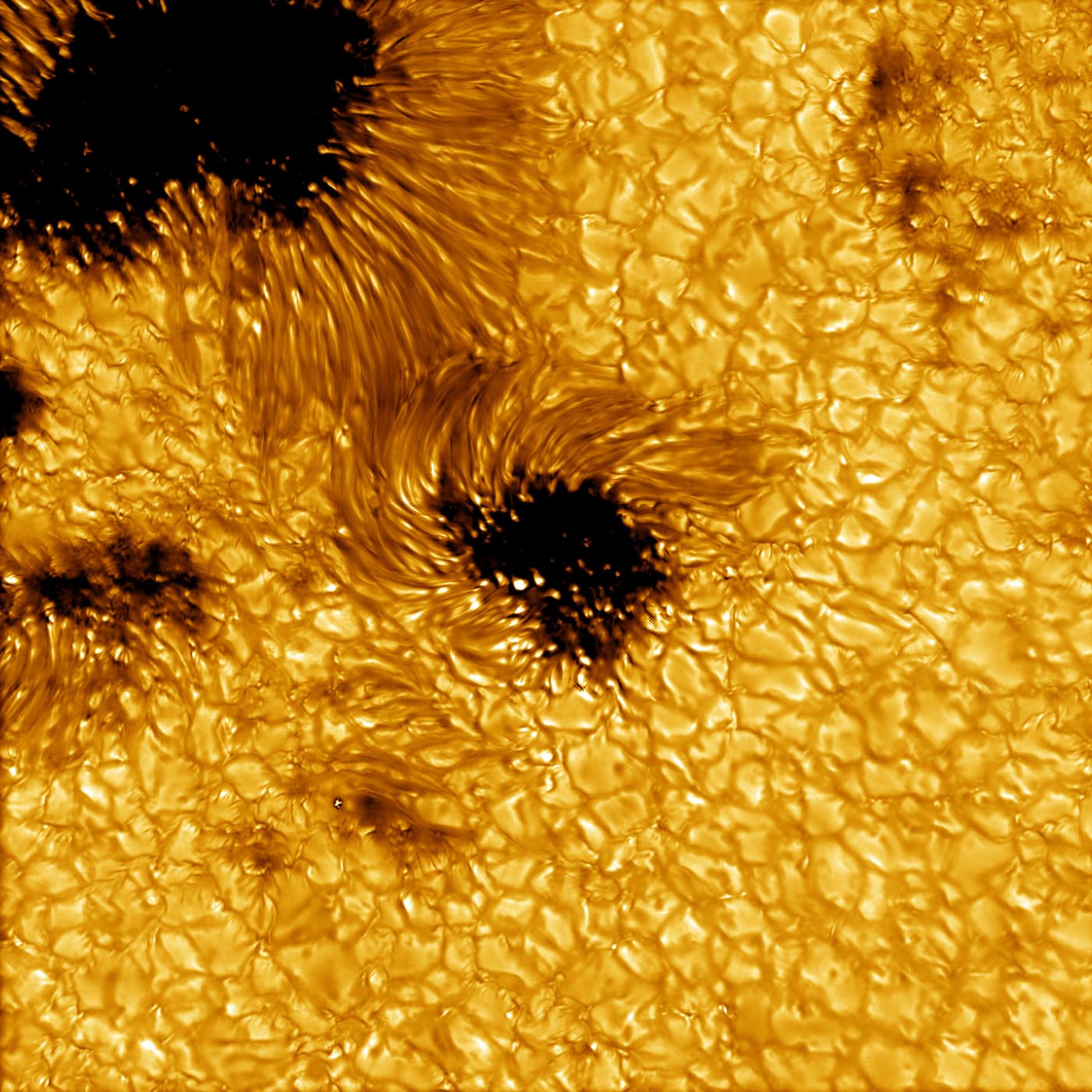This image presents a highly detailed and zoomed-in view of what appears to be an organic surface, possibly resembling the textured center of a sunflower or a similar flower. The predominant colors are a warm golden-yellow reminiscent of honey, interspersed with black spots, particularly noticeable towards the top left corner. These black spots are accentuated by flat, petal-like structures radiating from them. The entire composition is rich in texture, exhibiting a kernel-like effect across the surface. The image could plausibly depict something under a microscope, revealing the intricate, divided patterns and bubble-like formations that add to its complexity. Despite its unclear resolution, the visual suggests a natural, organic material, maintaining an overall impression of a golden mass interspersed with darker areas.